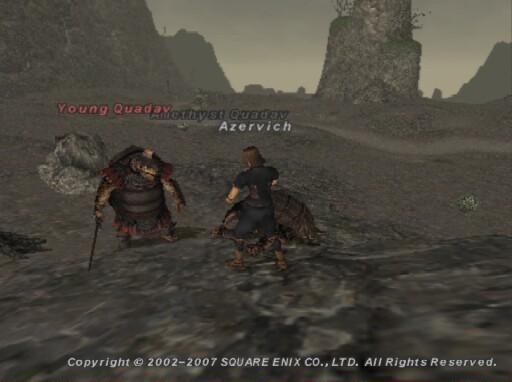This detailed screenshot from an in-game video game depicts two characters engaged in a face-off in a rugged, sparsely vegetated terrain. The landscape features gray dirt, hilly terrain with large boulders, and distant cylindrical mesa-like mountains under a lightly colored sky. The humanoid turtle creature on the left, named Young Quaday or Q-Day, is holding a sword. The human character on the right, named Amethyst Azervich, is dressed in a dark blue vest, pants, and leather boots. The scene is framed by text overlays: “Copyright 2002-2007, Square Enix Company, LTD, All Rights Reserved” in the bottom corner, and character names in white and red text. The characters, wearing armor and armed with weapons, are poised for combat on a slight rise in the terrain, standing out vividly against the desolate background.